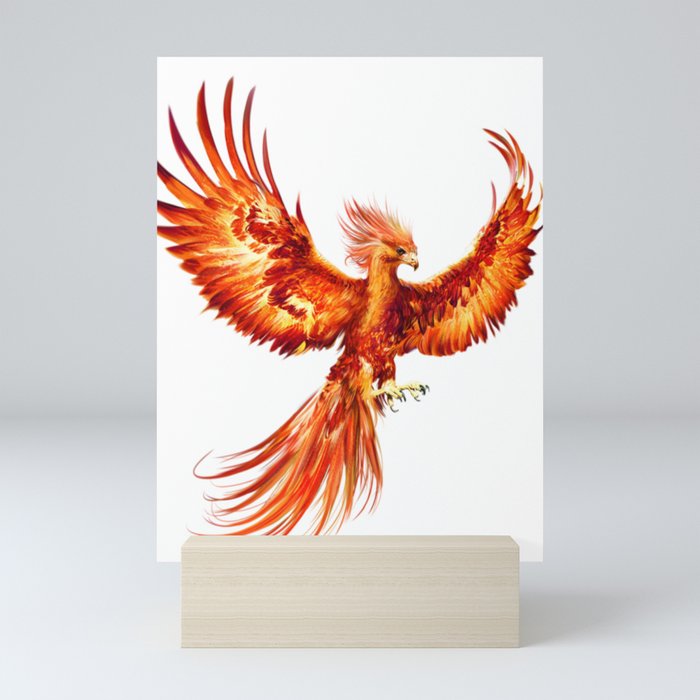The image depicts a striking phoenix-like bird adorned with fiery shades of red, orange, and yellow, appearing almost as if it's made of flames. Its wings are outstretched expansively to the sides, reaching the edges of the white backdrop, giving the impression of grandeur and power. The bird stands upright with its long, flowing tail composed of numerous feathers cascading in different directions, contributing to its majestic and dynamic presence. Its sharp feathers and talons, colored in yellow, add to its fierce and mythical aura. The phoenix's head and beak are also highlighted with bright, fiery hues. 

In front of the phoenix, there is a rectangular block of light tan wood with a horizontal grain, seemingly not interacting with the bird but adding a grounded element to the composition. The entire scene is set against a white background for the bird, which transitions to a gray backdrop for the rest of the image, enhancing the contrast and making the vibrant colors of the bird stand out even more. The overall artwork has a fluid and ethereal quality, capturing the essence of a phoenix rising from the ashes.